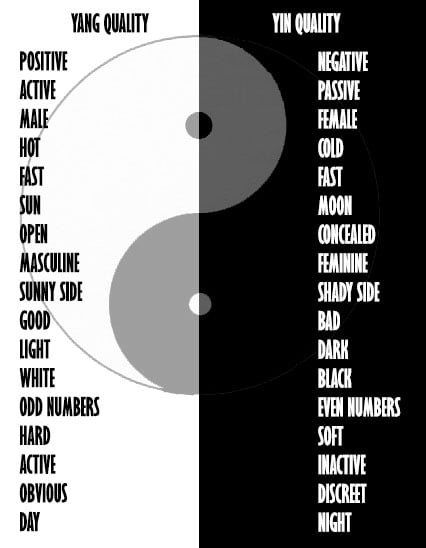This image prominently features a classic yin and yang symbol, encapsulating the dual nature of existence. On the left side of the image is the yang aspect, represented by a white semicircle, while its counterpart on the right side, the yin, is depicted by a black semicircle. 

Each side contains a list of adjectives that further elaborate on their intrinsic qualities. The yang side, marked by a central white field, has black text that describes attributes such as "positive," "active," "male," "hot," "fast," "sun," "open," "masculine," "sunny side," "good," "light," "white," "odd numbers," "hard," "active," "obvious," and "day."

Conversely, the yin side, symbolized by a deep black field, hosts white text detailing characteristics such as "negative," "passive," "female," "cold," "slow," "moon," "concealed," "feminine," "shady side," "bad," "dark," "black," "even numbers," "soft," "inactive," "discreet," and "night."

The contrast between the black text on the white yang and the white text on the black yin serves to emphasize the interwoven yet distinct nature of these opposite but complementary forces. This detailed visual and textual representation holistically illustrates the fundamental principles of balance, duality, and harmony in the universe.